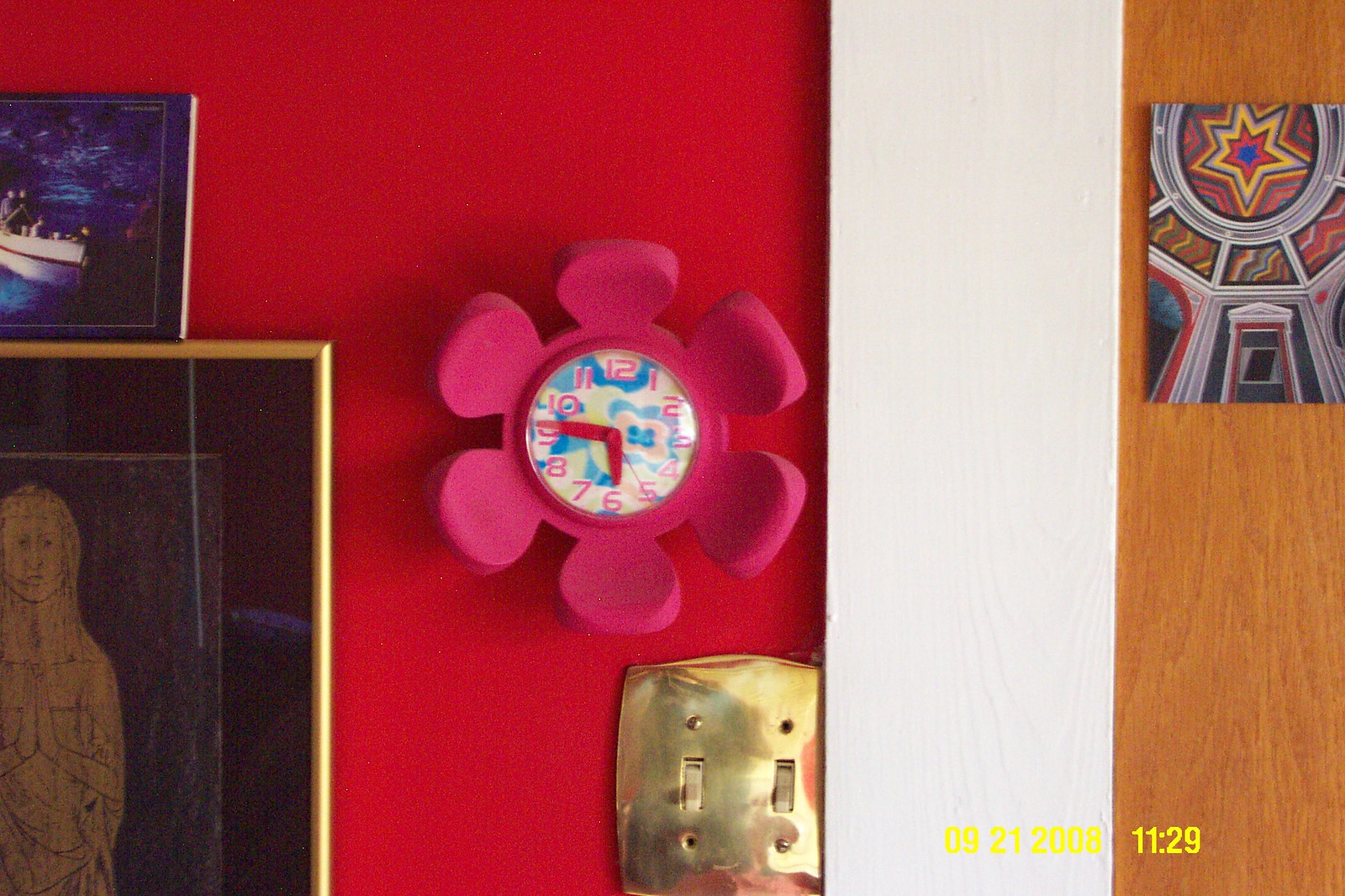This timestamped digital photograph, taken on September 21, 2008, at 11:29 AM, captures a brightly lit child's room featuring a vividly eclectic decor. The focal point of the image is a psychedelic, hot pink plastic flower clock with yellow, pink, and blue stylized petals, displaying the time as 5:45 with red hands. The background wall behind the clock is a striking lipstick red, adding to the vibrant atmosphere of the room. Adjacent to the clock are dual white light switches set on a shiny gold plate. 

The wall itself is divided into three sections: the dominant deep red portion, a narrow strip of white, and a tan wooden panel on the far right. The eclectic decorations include two framed artworks. On the left side of the red wall, one frame houses an older, stylized person or Virgin Mary-like figure, possibly in black and gold. Above it, there is a picture of a gray ship floating on water, set against a purple background. Finally, a hand-painted photograph in the wooden section features vivid colors—red, green, blue, and yellow—depicting a star atop a building with white walls, as if viewed from below.